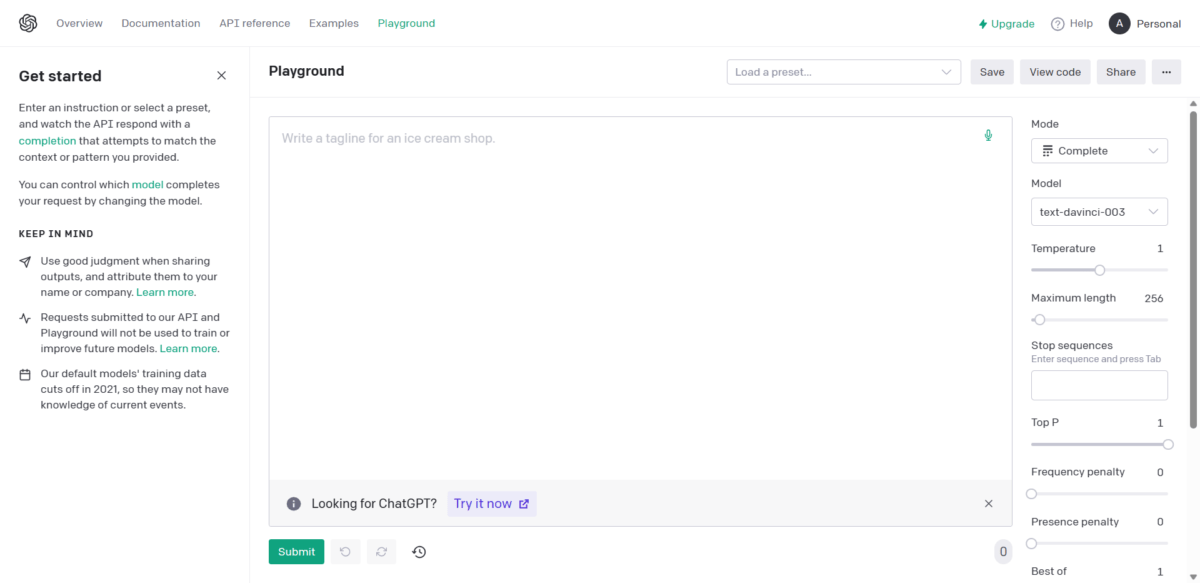A screenshot of the ChatGPT Playground interface, depicting a clean, minimalist design with a white background and black text accented by green hyperlinks. At the top, there's a navigation menu featuring the options: Overview, Documentation, API Reference, Examples, and Playground, with Playground being highlighted to indicate the current page. On the right side of this menu, there are buttons labeled Upgrade, Help, and Personal. The left-hand sidebar displays a "Get Started" section, which includes brief instructions for using the Playground. On the right-hand sidebar, users can configure various settings, such as selecting modes and adjusting text length. Dominating the center of the interface is a large text input field designed for user interaction.